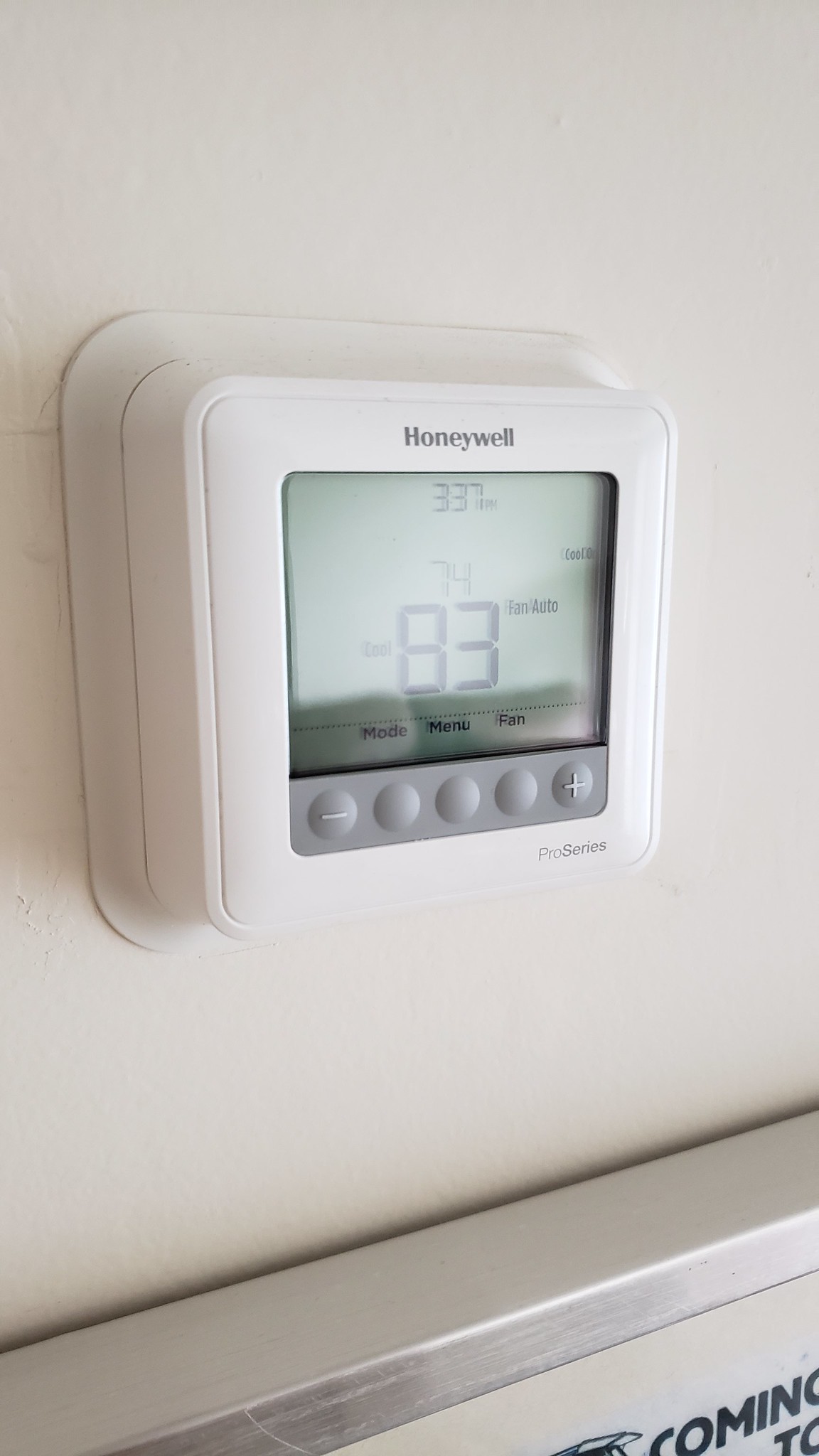This detailed photograph showcases a Honeywell Pro Series thermostat mounted on a pristine, white wall. The thermostat itself is also white, blending seamlessly with the background. The display reads 3:37 p.m., with the current room temperature at 83 degrees Fahrenheit. It is set to cool the room to a target temperature of 74 degrees Fahrenheit. The device is currently in 'cool mode' with the fan set to 'auto mode'. 

On the thermostat's interface, you can find various control buttons at the bottom, including those for mode, menu, and fan settings, alongside a plus (+) and minus (-) button for adjusting the temperature. Below the thermostat, a silver-colored metal ledge provides a subtle contrast to the overall white aesthetic. There is some partially visible text beneath this ledge, starting with "coming to," but the rest is obscured. The top of the device clearly displays "Honeywell Pro Series," affirming the model and make of the thermostat.